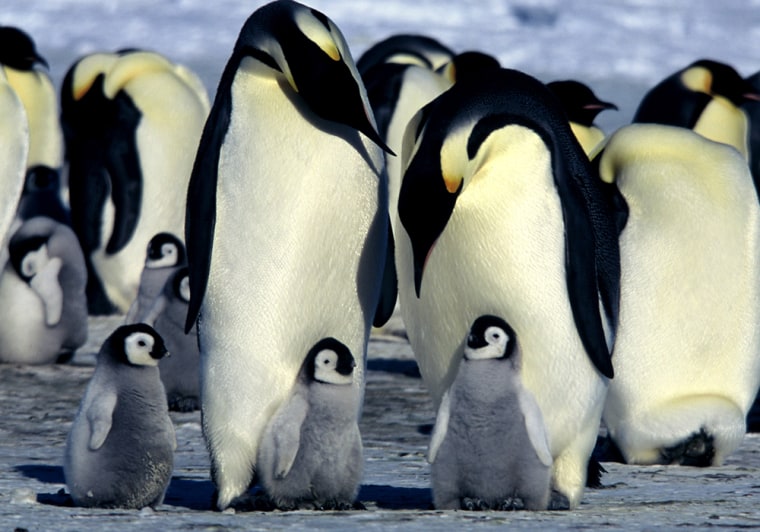This adorable photograph features a large group of Emperor penguins and their fluffy, endearing chicks, all gathered on a snowy expanse. In the foreground, two adult penguins, characterized by their striking black and white plumage with delicate yellow accents on their heads, are standing protectively over their three chicks. The adults gaze affectionately at their young, one of the chicks returning the gaze upwards. Surrounding them, there are additional adult penguins and six visible chicks. The baby penguins, significantly smaller than the adults, are covered in various shades of gray down, with their heads displaying a mix of black and white markings, adding to their charm. Their bodies appear plump and fluffy, distinct from the sleek appearance of the adults, and they stay close to their parents. The icy background, somewhat muted and grayed out, serves as a serene backdrop for this heartwarming scene of penguin family life. Some of the adult penguins in the background have their heads tucked back as if napping, creating a peaceful and endearing tableau.